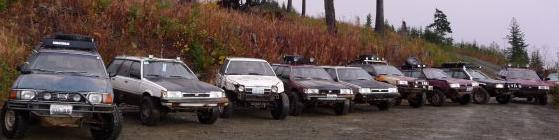In this landscape-oriented photo, there are nine modified older Subaru vehicles parked side by side on a gray concrete parking lot. The cars are arranged in a single line running parallel to a small hillside in the background, which is covered in a mix of brown and green grass. The vehicles, all appearing to be semi-wagons on raised wheels, showcase a variety of colors: a leftmost light blue car, followed by a white car with a black hood, another white car with large wheels, a black car, a gray and black car, an orange and red car, a purple-tinted car, another black car, and finally, a purple car on the far right. The scene is set against a field with light brown and green hues, with a few scattered trees visible in the distance and smaller trees on the right-hand side. The sky above is overcast and gray, contributing to the overall muted tones of the setting.